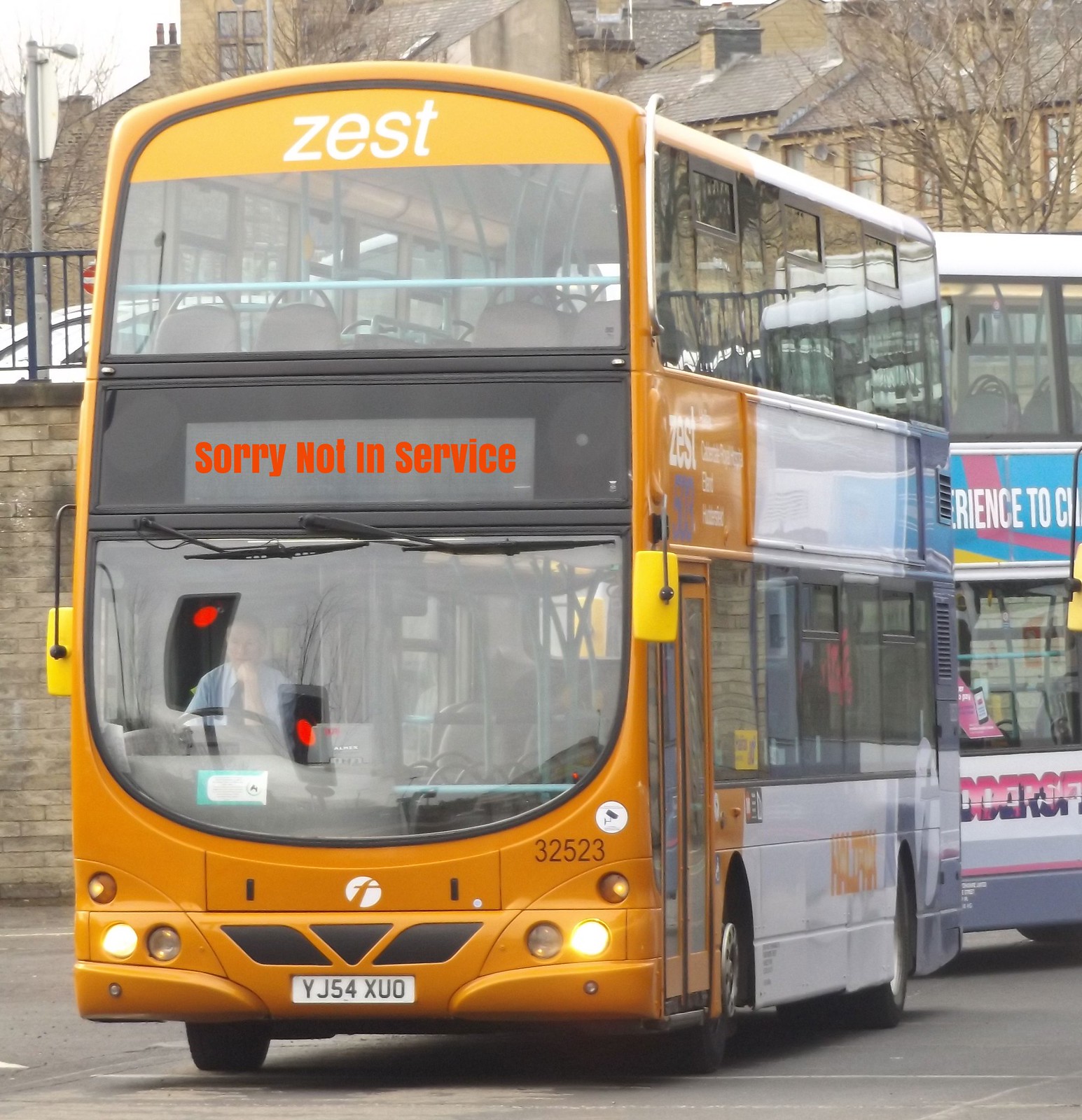The image captures a tall, striking double-decker bus with a bright orange front and sizable windows on both its lower and upper levels, providing clear views of the rows of seats inside. A person is visible in the driver's seat. Prominently displayed on the front of the bus is the word "ZEST" in large letters, and a digital sign below it reads, "Sorry, not in service" in red. The bus features white sides with a gray trim towards the back and has a license plate number YJFXU0. Advertisements are visible on the side panels, although they are not clearly readable.

In the background, there is another double-decker bus partially obscured as it appears to be moving behind the first bus. This second bus, largely white, also carries advertisements, including one with blue, pink, and yellow colors featuring the words "Experience 2" partially visible. The scene is set outside against a backdrop that includes a brick wall and various low, brown-stone structures with brown roofs, suggesting a possible location in England. The overall atmosphere of the photograph is influenced by the cloudy weather, underlining the typical ambiance of the setting.